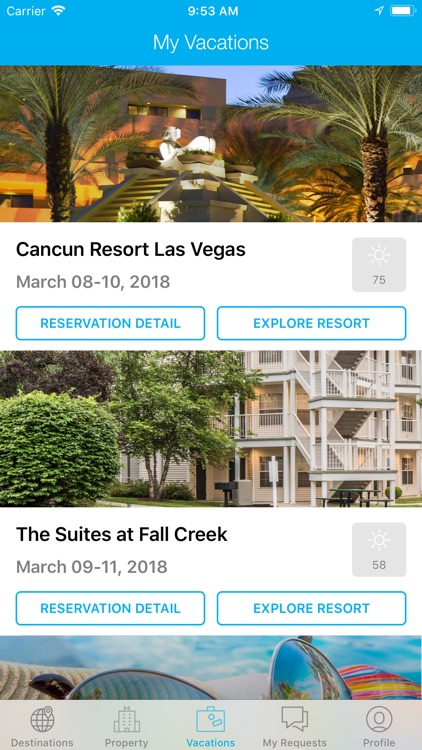Here is a polished and detailed caption for the image described:

---

The screen displays a vibrant travel application interface titled "My Vacations," highlighted by a blue banner at the top. Above the banner, the time reads 9:53 a.m., flanked by a nearly full battery icon at approximately 90% on the right, and a navigation arrow on the left. "Carrier" is displayed in white letters with a GPS signal icon beside it.

Prominently, the "My Vacations" heading reappears in white text against the blue background. Below this banner, a picturesque golden-lit resort image captures attention, showcasing palm trees on either side of a central Aztec-like step pyramid. A light, sand-colored cement building complements the pyramid in the background. Beneath the image, set against a white background, "Cancun Resort Las Vegas" is stated in black lettering, followed by the date range "March 08-10, 2018." On the right, a small gray square icon with a white sun and the temperature "75" in dark gray is displayed. Two buttons are below; "Reservation Detail" and "Explore Resort," both featuring a white background with blue outline and lettering.

Another image sits below, depicting a hotel or motel with outdoor access, visible doors and windows, external stairs with railings, and a picnic table in front. Trees flank the left of the structure. The caption reads "The Suites at Fall Creek," with the date range "March 09-11, 2018" in black lettering. Adjacent to this information is another sun icon displaying a temperature of "58" in dark gray. Similar buttons for "Reservation Detail" and "Explore Resort" are below the description.

At the bottom, a bright blue sky with minimal clouds is partially visible in a third image, obscured by a translucent gray banner with five icons. From left to right, these icons include:
1. A globe labeled "Destinations"
2. A building labeled "Property"
3. A blue-highlighted briefcase labeled "Vacations," emphasizing its current selection
4. Chat bubbles labeled "My Request"
5. A profile icon representing user profile access

---

This revised caption provides a clear, detailed description that enhances the visual context and functionality within the app screen.